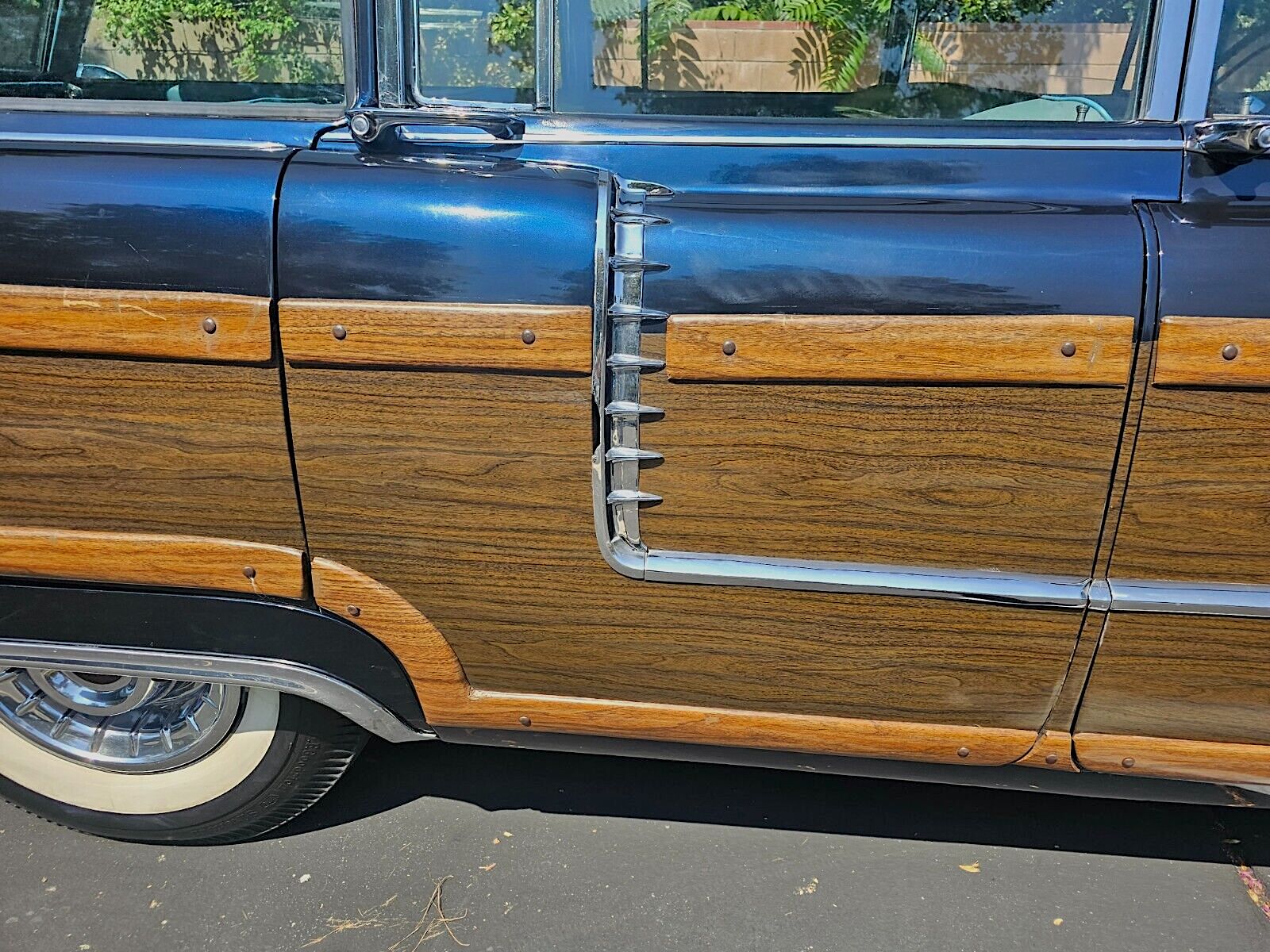The image depicts a side view of an old-fashioned station wagon-like car with a distinctive design. The vehicle features a dark blue upper section covering approximately one-quarter of the door, while the remaining three-quarters is adorned with pronounced wooden paneling, secured with visible screws. There are bullet-shaped metal hinges along the door, and the silver detailing is prominent throughout the car's trim. The wheel visible on the left side is partially obscured by a wooden and black fender, and it sports a black tire with a thick white stripe, complemented by silver rims. Sunlight shines on the car, emphasizing its blue and wood tones. Through the large windows, which are characteristic of an older style automobile, the light blue interior seats are faintly visible. The scene includes a backdrop consisting of a brick wall, scattered green leaves, and possibly a wooden fence with fern-like greenery, situating the car in an outdoor setting, taken during the daytime.